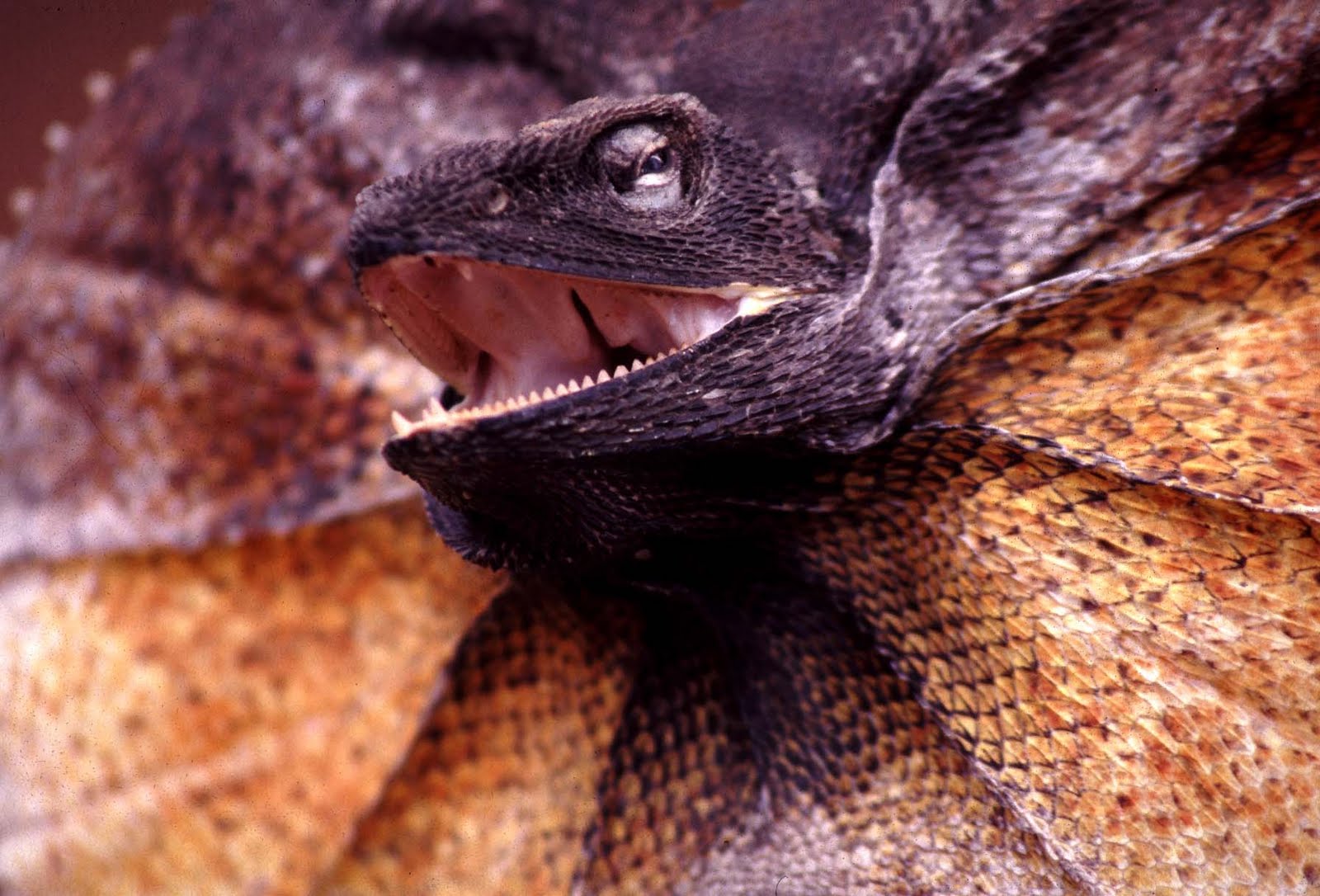This image features a detailed close-up of a reptile, prominently displaying its striking features. The focal point is the creature's large head with a purplish-black face and a pronounced, pointed snout. The reptile has a sizable eye positioned on the upper part of its face, encircled by white and gray scales. Its mouth is open, revealing small, sharp white teeth set against a pink interior and white lips.

The body of the reptile is adorned with an intricate pattern of scales in hues of black, brown, and white, extending from behind the head to the lower parts of the image. These scales form a complex design, with some sections displaying a tan or orangeish-yellow tint. The creature’s neck flares around the head, adding to its dynamic appearance, and the lower part of the neck showcases vibrant orangeish-yellow and black scales. The background of the image appears mostly gray, possibly with some indistinct objects or shadows.

The overall composition captures the reptile in a natural yet menacing pose, with its eye, imposing jaws, and textured scales as the primary elements, creating an evocative portrayal reminiscent of a prehistoric predator.